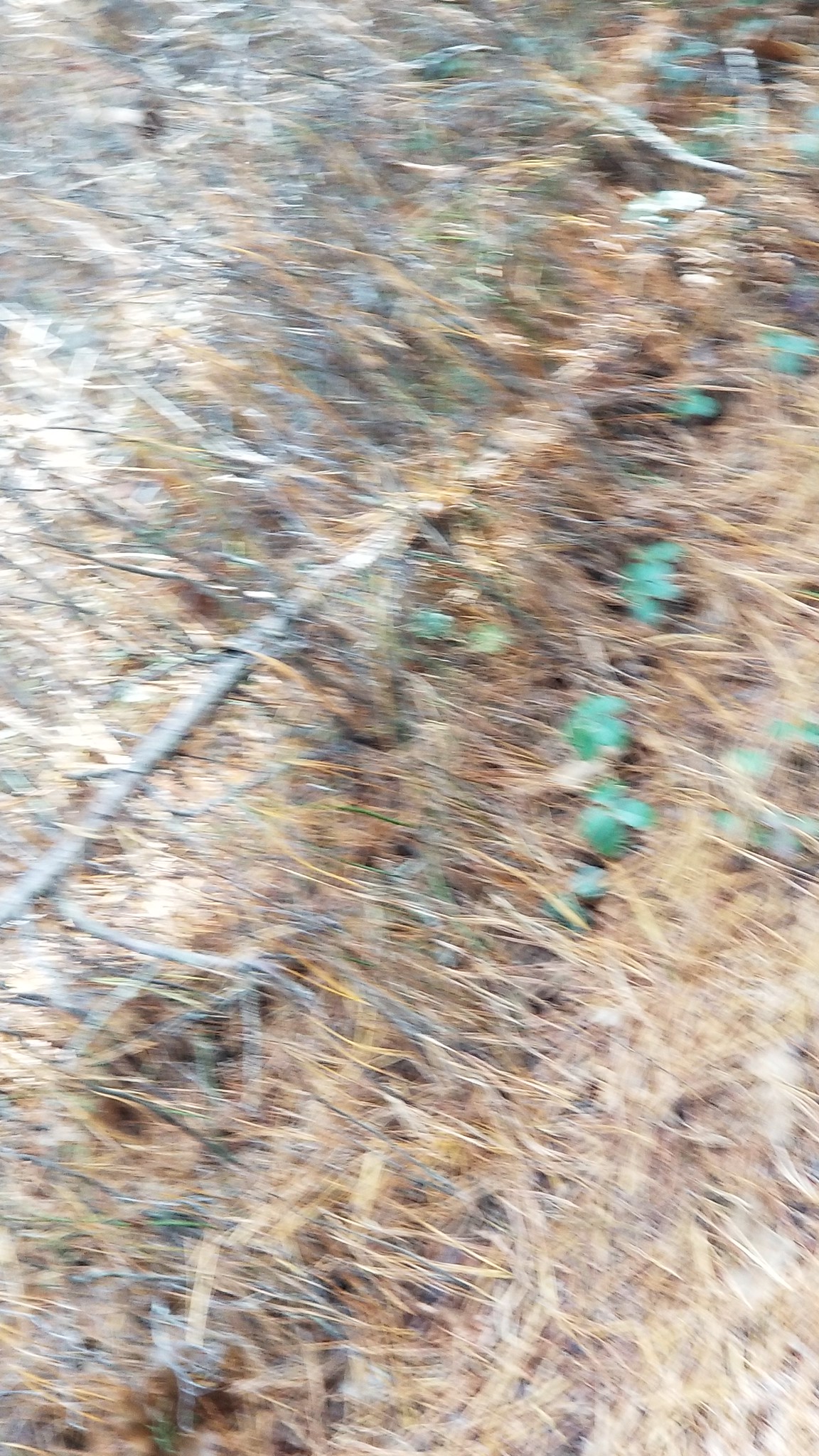This extremely blurry photograph captures a rather desolate outdoor scene, marked by dying vegetation and sparse greenery. The predominant colors are tan and brown, with gray and green elements interspersed throughout. Central to the image, there's a thin, gray tree branch extending diagonally from the left side towards the center, adorned with a few sparse, green leaves or small plants. Surrounding this branch are patches of brown grass and dried vegetation, giving the impression of a dehydrated or desert-like area. Small, dark green plants or weeds dot the ground, particularly in the right center and top right of the image. Additionally, lighter green grass can be observed from the bottom right extending slightly leftward. The landscape appears hilly and uneven, suggesting an area with little to no water, emphasized by the overall lifeless and dry appearance. Although it’s daytime, the brightness of the sun in the blurry photograph does not create any discernible shadows within the frame.